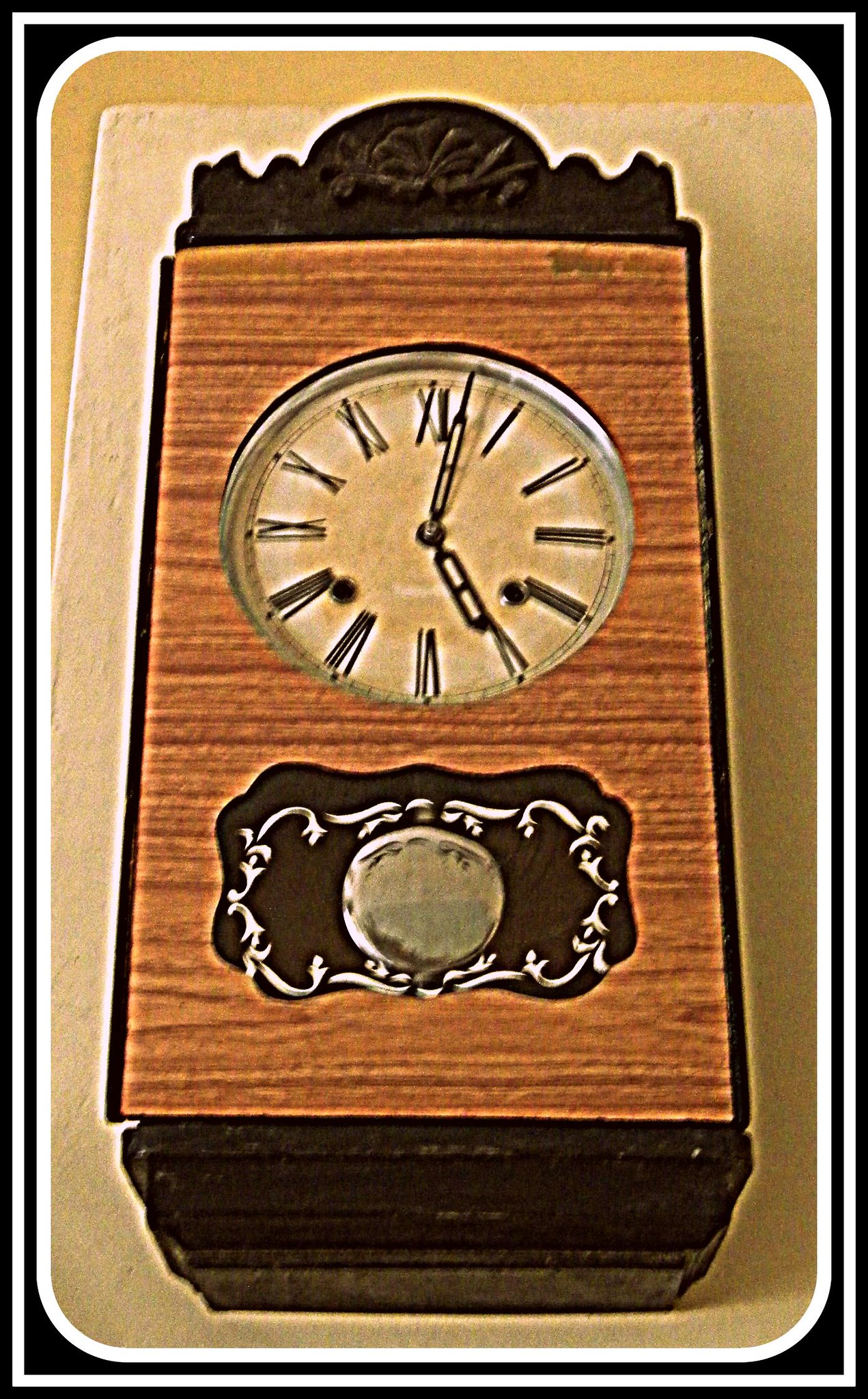The image is a grainy color photograph of a vertically rectangular clock with a series of ornate and detailed borders. The clock is framed within a poster-like design with several layers: an outer black border, followed by a white border, and another inner black border, all surrounding a parchment-colored background with curved corners.

The clock itself, which appears to be made of wood, has dark brown ornate woodwork at both the top and bottom, featuring scalloped and embossed designs. The central body of the clock is composed of light brown wood, showcasing the wood grain.

The clock face occupies the upper section of the clock structure and is distinctly aged in appearance, reminiscent of old ivory or parchment paper. It features large Roman numerals marking the hours, and the time displayed is approximately 5:02. The clock hands have decorative holes in them, adding to its antique aesthetic.

Below the clock face, there is a dark chocolate brown section with a squiggly, ornate border accented by white decoration. At the center of this section, a gold disc is visible, possibly part of a pendulum or decorative feature. The overall impression is of a vintage, carefully crafted timepiece encased in an elegant, layered border design.